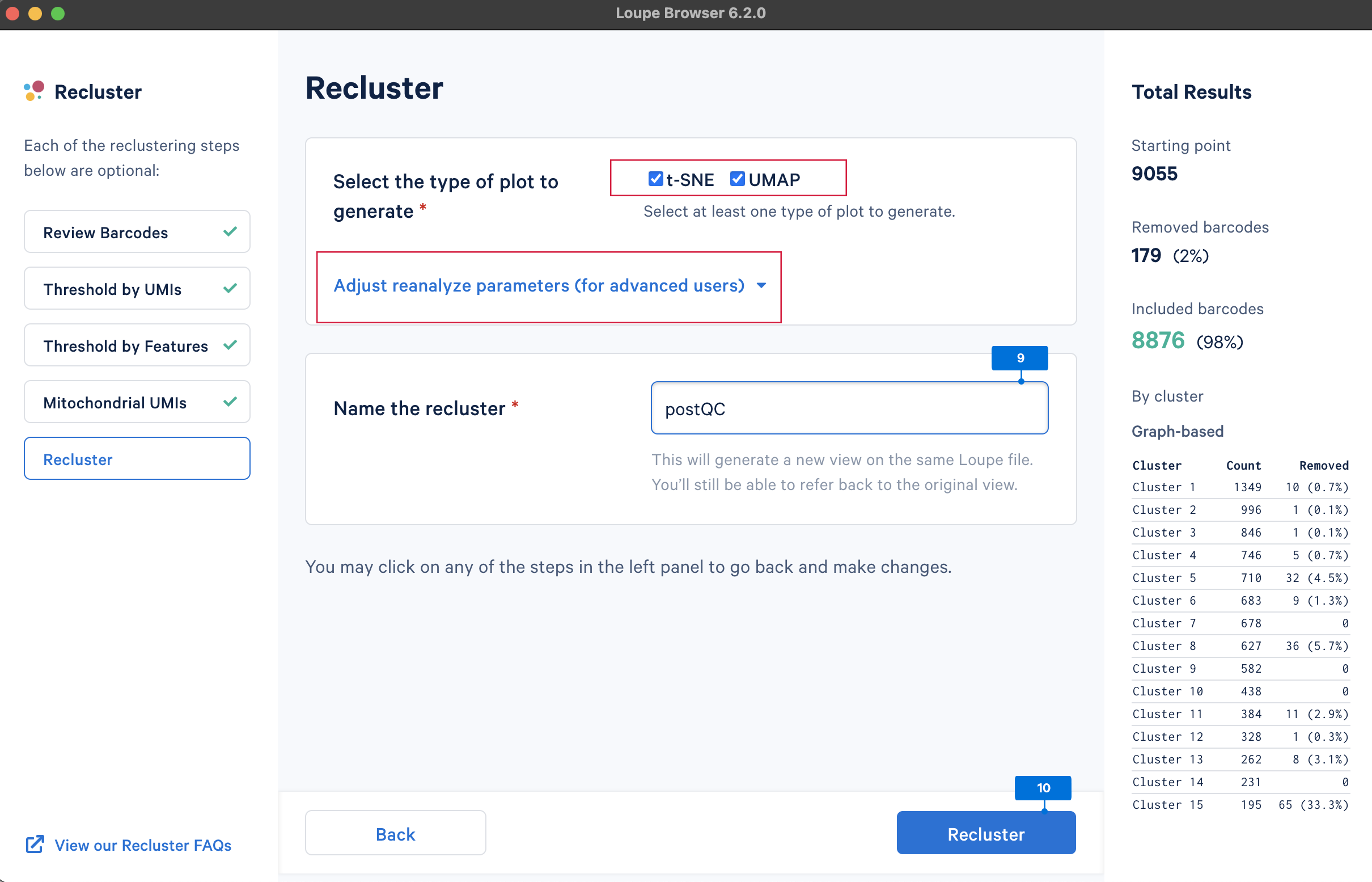The top section of the image features a long black bar that contains three small circles on the left side. The circles are color-coded: red, yellow, and green. To the right of these circles, in light gray text, the caption displays "LOUPE Browser 6.2.0."

At the center of the image, the word "Recluster" is prominently displayed. Below this, there is an instructional phrase: "Select the type of plot to generate." Adjacent to this instruction, two colored boxes offer plot options: "T-SNE" is within a red box with a checkmark inside, and "UMAP" is within a blue box, also with a checkmark inside.

Further down, a red box provides advanced options for users with the phrase, "Adjust/Reanalyze Parameters for Advanced Users." Nearby, there is a section to name the recluster operation, accompanied by a rectangular input field labeled "Post QC." This field comes with a note indicating that generating a new view will still allow users to refer back to the original view.

Additionally, users are informed they can click on any steps in the left panel to revisit and make changes.

On the right side of the image, black text lists the total results, divided into different categories. The "Starting Point" is 9,055. "Removed Barcodes" total to 179, which is 2% (indicated in parentheses). The remaining "Included" results are 8,876, equating to 98% (in parentheses), and this data is shown in green. The caption concludes with the phrase "By cluster," followed by "graph-based" to indicate the type of clustering method used.